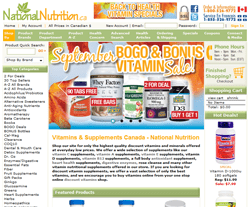The image displays a website named National Nutrition, distinguished by a small leaf icon located in the upper left-hand corner. Across the top of the page, a heading reads "Back to Health Vitamin Specials". The text throughout the website is generally blurry and challenging to read. The central visual feature is a grouped display of various vitamin brands, overlaid with a promotional message in orange text stating "September BOGO and Bonus Vitamin Sale." Additional images on the page show various bottles of vitamins.

The site also includes supplementary text, though most of it reads indistinctly due to the blurriness. One noticeable banner with a green background and white text is particularly illegible. On the right-hand side of the page, a column displays an orange telephone icon accompanied by the title "Phone Hours" followed by more blurred text. Below this section, there is an orange shopping cart icon labeled "Finished Shopping Checkout". Further down, it mentions "Shopping Cart" with additional unreadable text. The bottom right corner of the page features an image of another vitamin bottle with more obscure text next to it. 

Overall, the page seems focused on promoting vitamin specials and sales, though much of the specific details are lost to the poor image clarity.